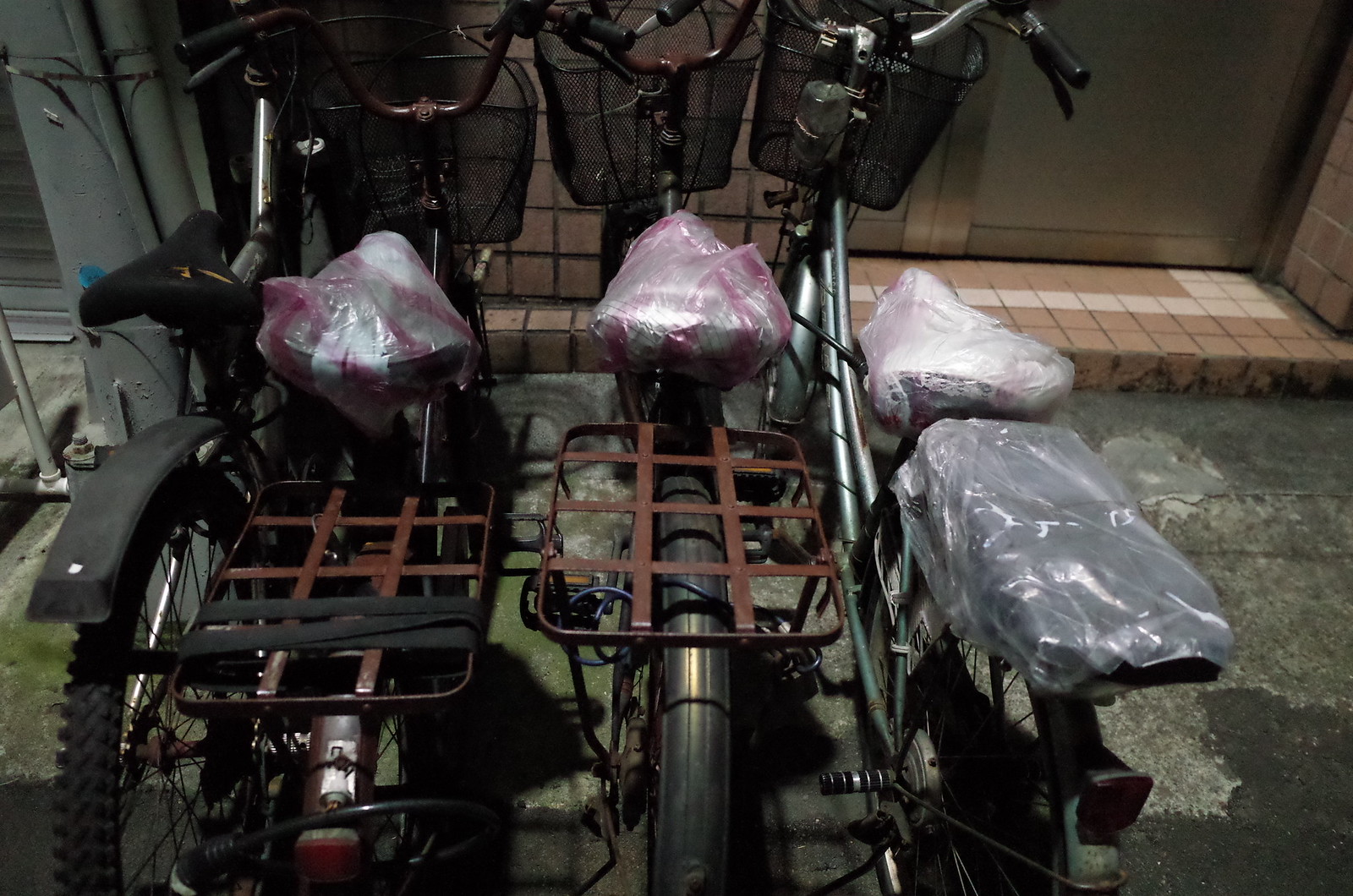The image depicts a set of four bicycles parked in a warehouse-like setting. The three main bicycles, which are centrally positioned and facing a brick-style wall composed of small squares, are the focal point of the scene. These bicycles have large wheels and are equipped with metal racks at the back for cargo, which are visibly flat with straps for securing items. Each bike also features a front basket for additional storage. The seats on these bicycles are wrapped in plastic, possibly for weather protection. Notably, the bicycle furthest to the right has a slightly more elaborate design, including an extra cushion on the rear rack, potentially for passenger seating, along with footrests. In the left corner of the image, a partial view of a fourth bicycle can be seen, blending into the background. The setting appears somewhat worn down, hinting that it might be in a less affluent area.